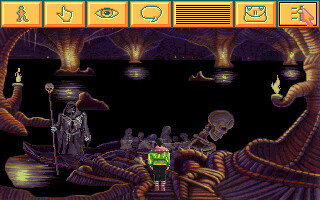This is a small, rectangular screenshot from an old-fashioned, vintage video game or computer game. The image features a man in the center, dressed in a green long-sleeve shirt with yellow accents, and he has a large cowl or scarf around his neck that is red with yellow dots. He has short black hair and is wearing boots. The man is standing on a dark, bone-like walkway that has rounded, brown sides and steps. To the right of the man, there is a large skeleton and a faceless demon-like figure in a black cloak, carrying a staff topped with a skull. The setting appears to be an underworld or underground environment, with dark and eerie elements. At the top of the screen, there are seven yellow square buttons. The first button features a silhouette of a person, the second a pointing hand, the third an eye, the fourth a speech bubble, the fifth vertical black lines, the sixth a bag or purse, and the seventh has a red arrow over it.